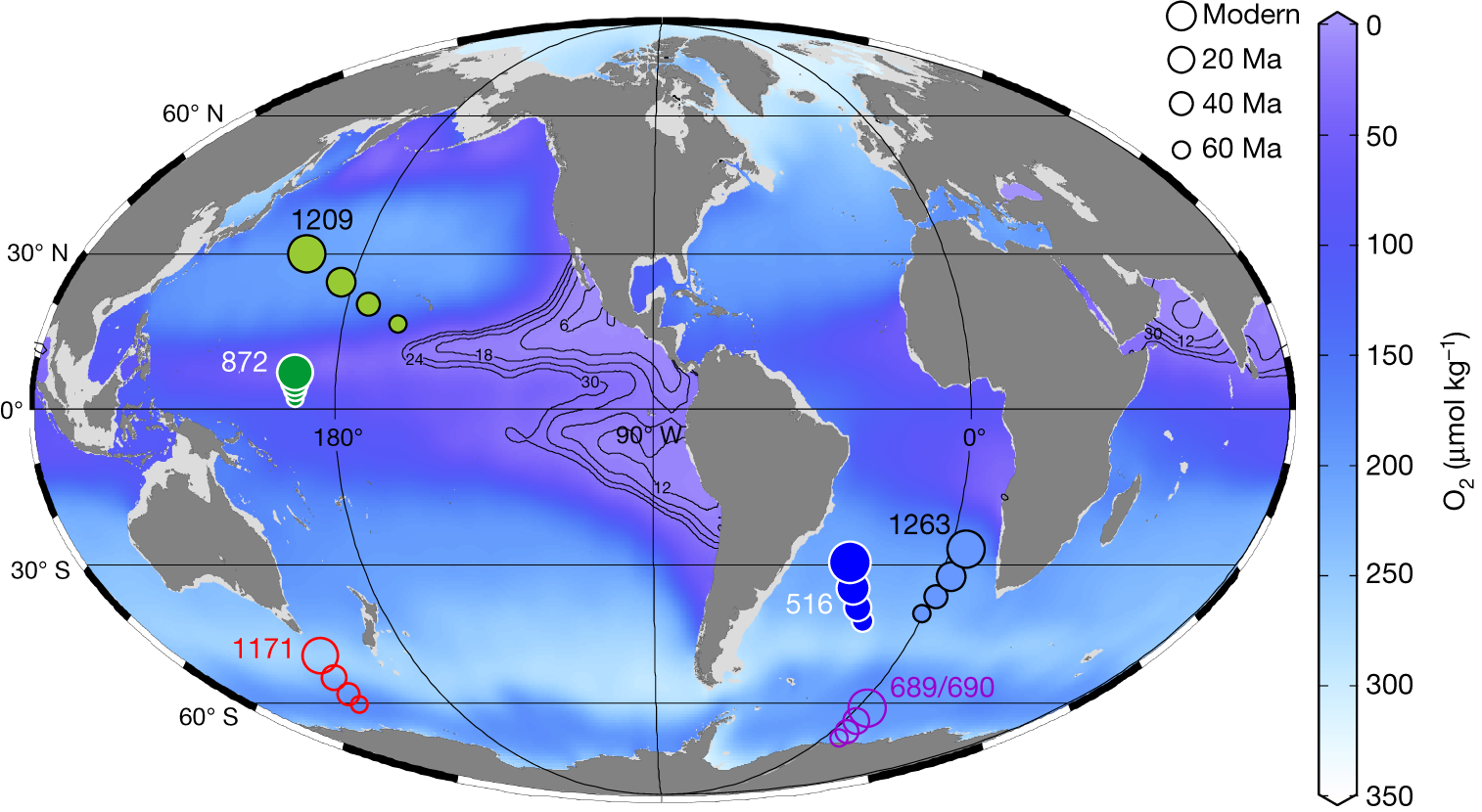This image is of an oval-shaped world map with detailed geographical and scientific notations. The landmasses on the map are depicted in shades of dark grey and light grey, while the bodies of water are illustrated in blue. Along the left side of the map, there are degree markings indicating latitude: starting from 60°S at the bottom, moving up through 30°S, 0° (equator), 30°N, and reaching 60°N at the top. The left side of the map prominently features Asia and Australia, while the central portion depicts North and South America, including the United States, Mexico, Canada, and Greenland. Europe and Africa are located on the right side.

On the right side of the map, there is a vertical scale labeled for O2 concentrations, measured in micromoles per liter (µmol/L). The scale starts at 350 at the bottom and ascends to 0 at the top, with a gradient transitioning from white at the bottom to purple at the top. Additionally, there are four green circled dots positioned to the left of the globe.

At the top right of the map, there is a section with the word "modern" situated near a sequence of three circles. Each circle is labeled with black text indicating different timescales: "20ma," "40ma," and "60ma." The map is bordered by alternating black and white sections, adding further detail to its perimeter.